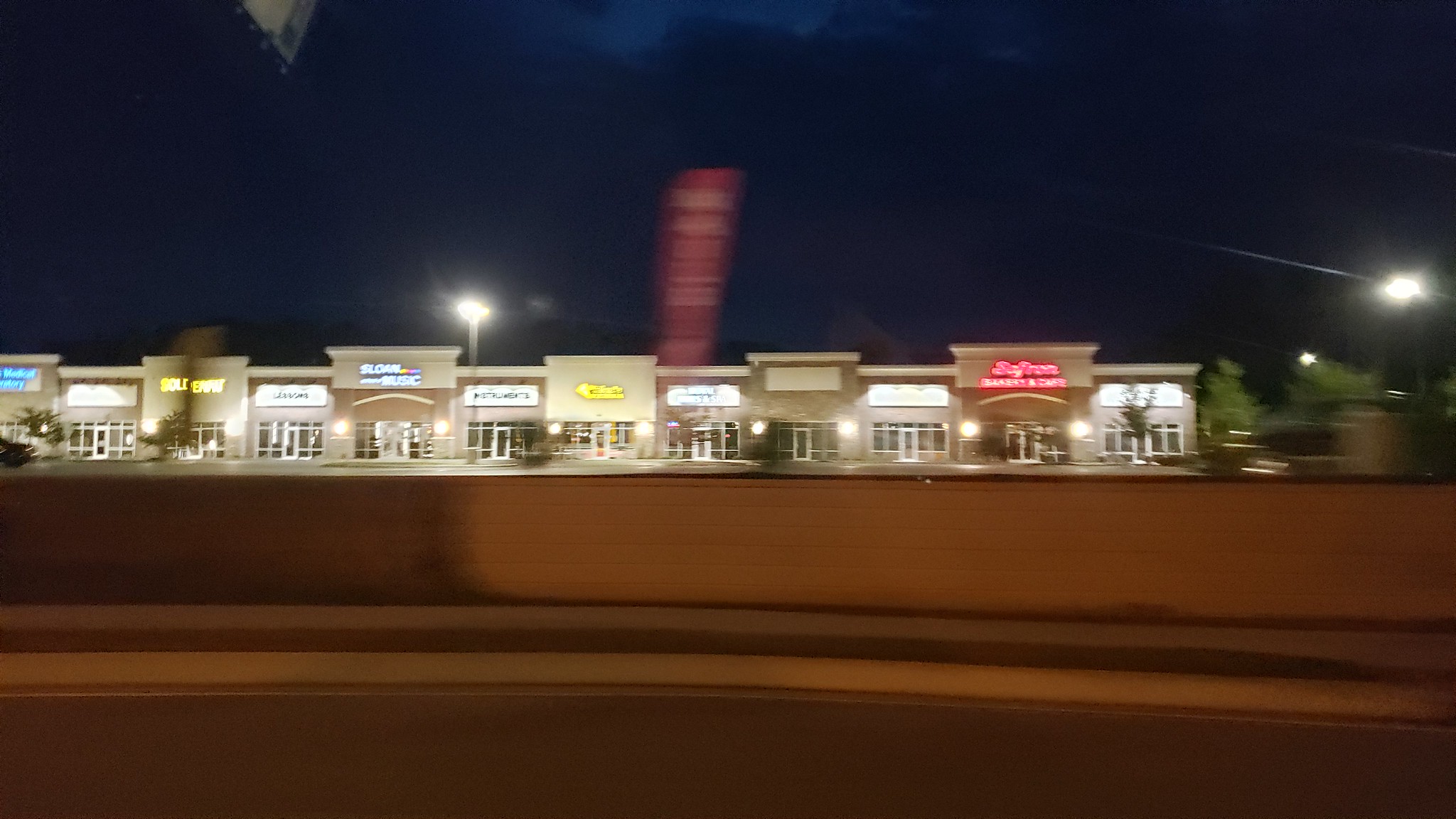This blurry nighttime image, captured from a moving vehicle, showcases a stretch of various businesses in a shopping center set against a deep midnight blue sky. The shopping center features multiple neon-lit signs in hues of blue, yellow, white, and red, illuminating the surroundings. Dominating the center of the photo is a tall, narrow, rectangular red flag with indistinguishable white lettering. Running parallel to the shopping center, there's an empty parking lot followed by a concrete barrier and an adjacent roadway. In the foreground, a segment of the sidewalk and a slender concrete block are visible. Toward the top left of the image, part of a billboard or road sign is seen hanging over the roadway, while the right side of the image is illuminated by a distant street lamp. Scattered trees are interspersed among the storefronts, adding a touch of greenery to the scene.